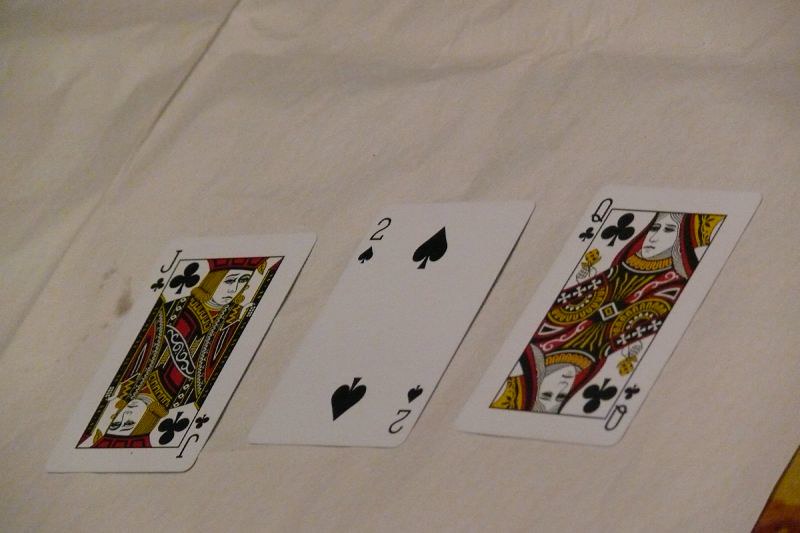In the image, three cards from a standard deck are meticulously arranged on a pristine white piece of paper, which rests atop what appears to be a brown wooden table—evident from the visible lower right corner of the image. The three cards, positioned from left to right, are the Jack of Clubs, the Two of Spades, and the Two of Clubs. 

The Jack of Clubs features a character adorned in royal attire with strikingly colored garments in yellow, red, black, and white. This character, with yellow hair, is depicted in a symmetrical, mirrored design that spans the vertical axis of the card. Similarly, the Queen of Clubs—although the initial description mistakenly refers to a Queen that is actually not pictured—would traditionally share the same coloring and regal aspect.

The remaining cards are the Two of Spades and the Two of Clubs, each showcasing their standard symbolic representations in black on a white background. Both the Jack and the two numbered cards exhibit minimalistic yet classic playing card designs.

The overall scene is absent of any legible text, emphasizing the simplicity and elegance of the playing cards against the white paper and the contrasting wooden surface.